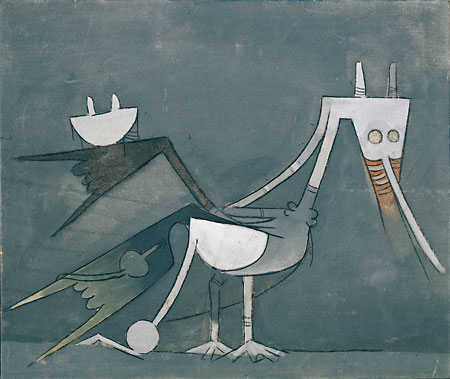This image is a modern, stylized illustration of a very strange-looking, abstract bird standing on a ground that seamlessly blends into a gray background. The bird, facing to the right, has an upside-down triangular head adorned with two straight horns and two rounded tan eyes. The creature possesses an orange and yellow beak with a long, white mosquito-like protrusion extending from the nose area. Its thin neck leads to a gray bird-like body supported by two legs with webbed feet. 

Behind the bird, there are two sets of wings; the upper wings are dark gray verging on black, featuring what appears to be a bowl-shaped object, while the lower wings feature a gradient from light to dark gray or even green and have sharp, pointed ends. The bird's tail ends in a large ball, adding to its peculiar appearance. The overall style of the illustration combines areas that resemble pencil sketches with more fully colored sections, giving it a unique, creative feel.